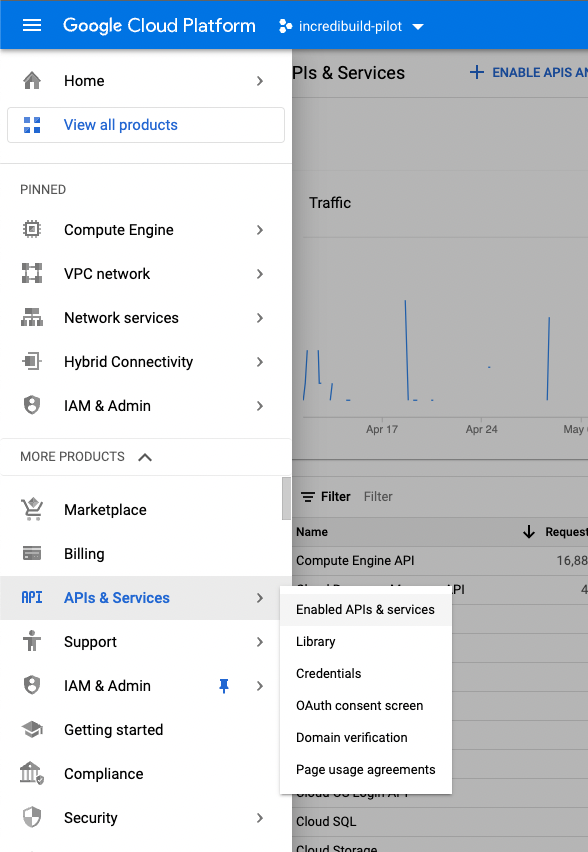This image from the Google Cloud Platform website prominently features the "IncrediBuild Pilot" dropdown menu displayed at the top in blue. Below it, "Home" and "View All Products" are also highlighted in blue. The screen is divided into two sections. The left side, which is white, features sections titled "Pinned" and "More Products." Under "Pinned," different categories are listed, and under "More Products," additional categories are displayed, with "APIs and Services" highlighted in blue. This section brings up a pop-up box containing options like "Enabled APIs and Services," "Library," "Credentials," "OAuth Consent Screen," "Domain Verification," and "Page Usage Agreements." 

An actual blue pin icon is shown, pinning the "IAM and Administration" section. The right side of the split screen is gray and appears to be incompletely captured, showing only the middle portion of a page. This gray area contains partial information, such as "Enable APIs and," which is cut off and mentions a term "Traffic" in black. Dates such as "April 17th," "24th," and "May something" are visible but incomplete, making this side of the screen less informative.